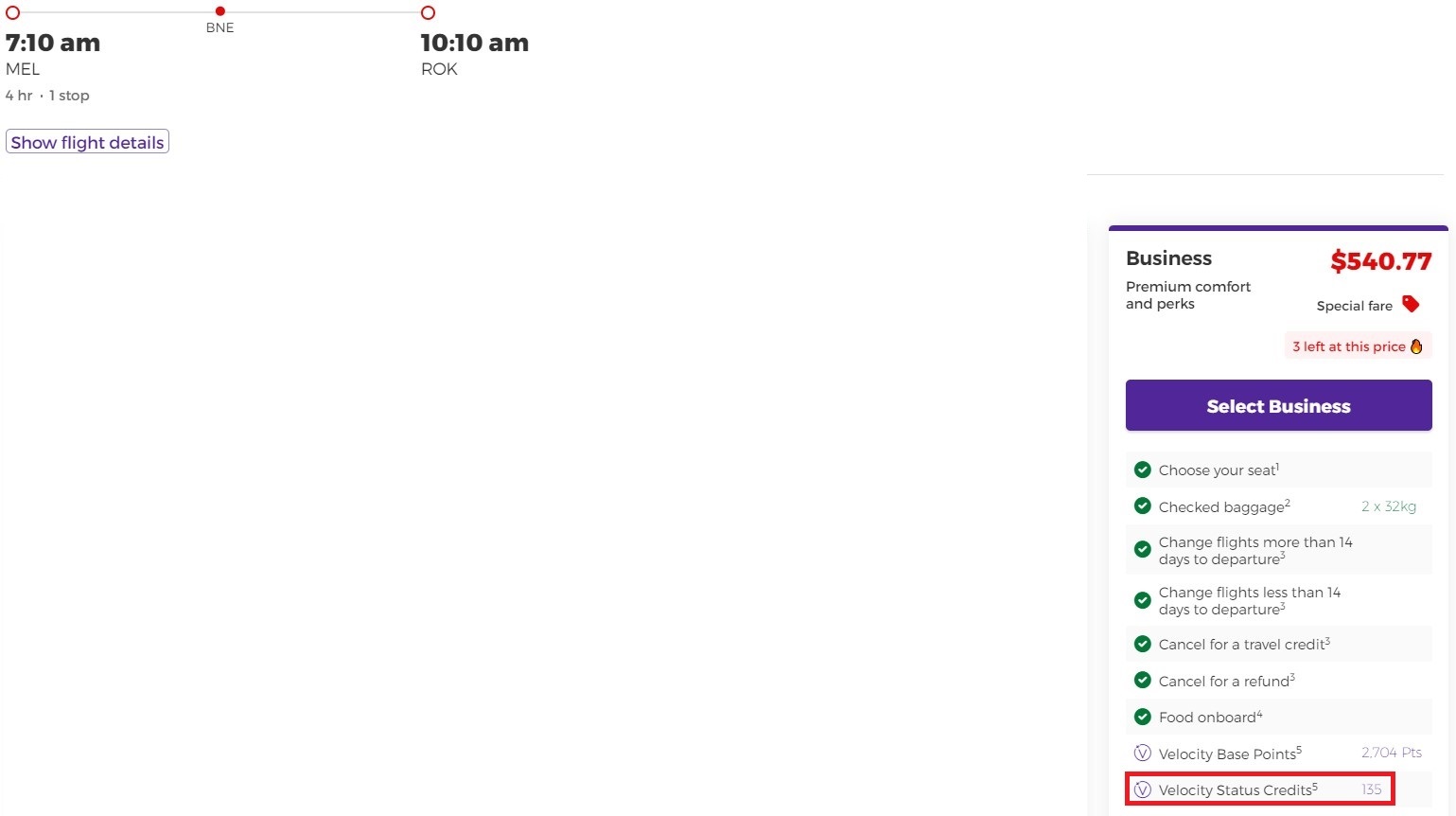Caption: 

An intricate image showcasing various flight and fare details, with several sections of overlapping text and information. In the upper-left corner, a band featuring small red dots indicates a time of 7:10 am and a location label "Mel." Additionally, there is a 4-kilometer metric and a notation of "one stop." The same section also displays "10 am" on the right and a term that looks like "FROK." Below, a box labeled "Show Flight Details" is present in white text.

The central part of the image prominently features "B&E." On the bottom right, another screenshot appears to be superimposed, overlaid with a blue band labelled "Business" and a fare amount of "$540.77" in red. Below, a section titled "Premium Comfort and Perks" highlights a "Special Fare" with only three seats left at this price. 

A purple box with white text underneath invites the viewer to "Select Business." The next section lists several options in black text with accompanying green checkboxes: "Choose your seat," "Checked baggage, 2 x 32 kg," "Change flights more than 14 days before departure," "Change flights less than 14 days to departure," "Cancel for travel credit," "Cancel for refund," and "Food on board," each with specific footnotes.

Additionally, "Velocity Base Points" is indicated with a 'V', showing 2704 points, and "Velocity Status Credits" marked with a '5', tallying up to 155. The "Status Credits" section is highlighted in a red box at the bottom of the image.